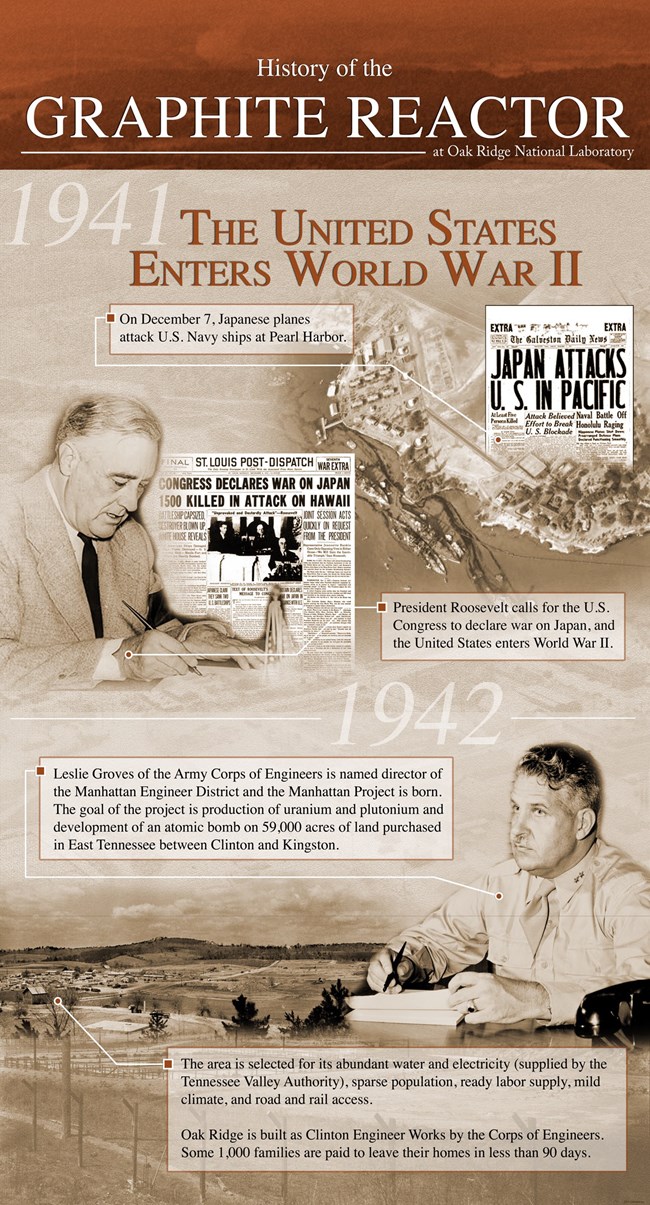The image is a detailed, color infographic illustrating the history of the graphite reactor at Oak Ridge National Laboratory. The top portion features a rust-colored band with white text that states, "The History of Graphite Reactor at Oak Ridge National Laboratory." Below this, on a tan background, the year "1941" is highlighted in white, followed by the phrase "The United States enters World War II" in orange-brown text.

The timeline starts in 1941 and is broken into chronological segments with text boxes providing key historical events. The first box notes the attack on Pearl Harbor on December 7, 1941, with a close-up of a newspaper headline reading "Japan Attacks U.S. in the Pacific," accompanied by an aerial photograph of Pearl Harbor. Following this, there is an image of President Roosevelt signing the Declaration of War against Japan with corresponding text.

Moving into 1942, the infographic continues with further details and events. A prominent box provides extensive information about the developments and significance of that year. To the right, there is a picture of Leslie Groves, identifiable by his military uniform with epaulets, and an image showcasing the site of the Manhattan Project, set against a backdrop of a valley with trees and a road.

The infographic is richly detailed with both text and photographs, creating a comprehensive visual narrative of the graphite reactor's history and its context within World War II.